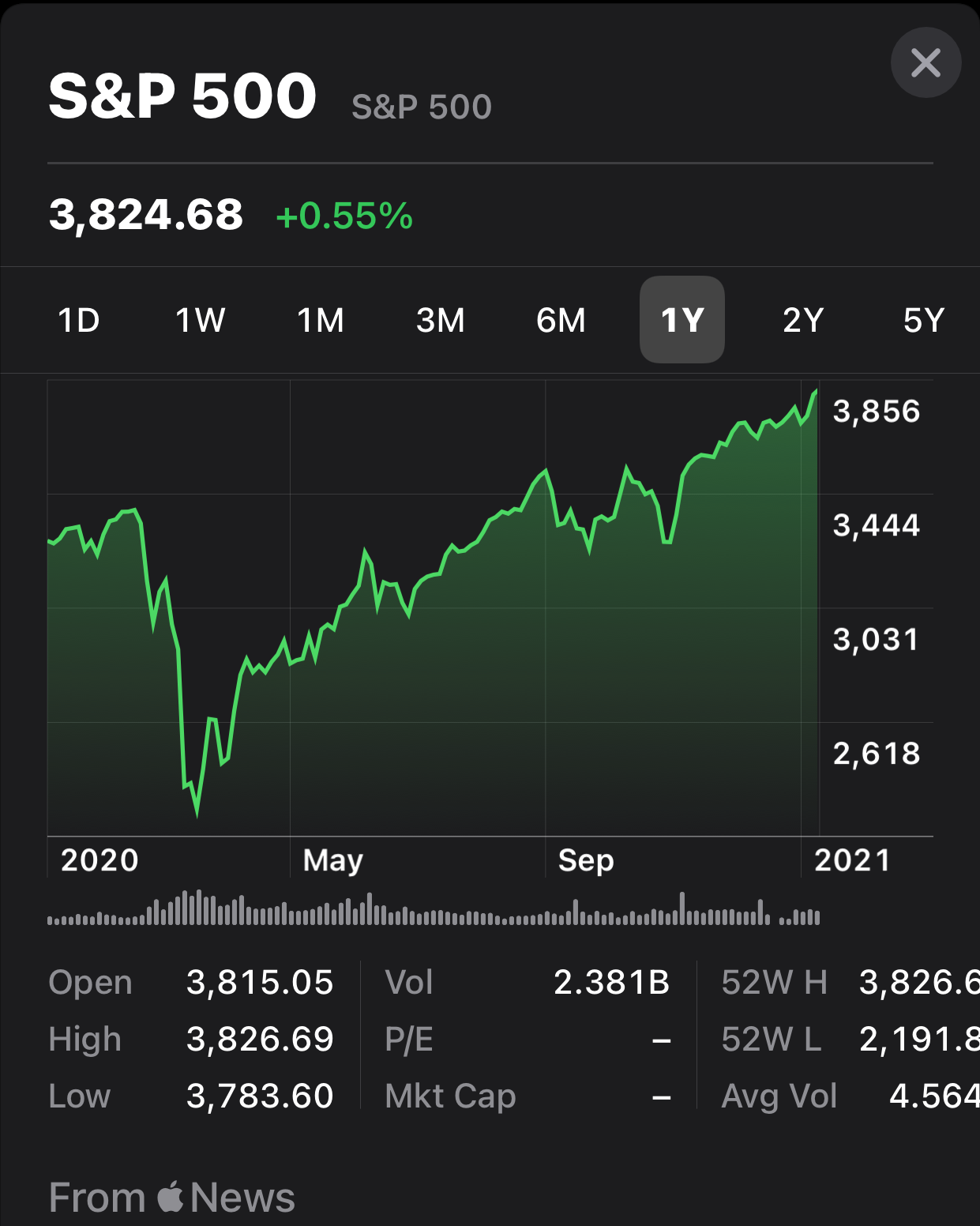A pop-up window is displayed against a black background, containing detailed information about the S&P 500 performance. The pop-up is identifiable by a small "X" in the upper right-hand corner, indicating it can be closed. At the top of the window, bold white letters spell out "S&P 500," with smaller off-white text immediately repeating the same. The main figure shown is "3,824.68," highlighting that the data is outdated as the current S&P 500 levels are significantly higher.

In green text, it denotes a significant increase of "55%" for the day. The predominantly white text is accompanied by a line graph shaded underneath in green. This graph offers the option to view data over various time frames, including one day, one week, one month, three months, six months, one year, two years, and five years. The "one year" option is highlighted, indicating the graph shows the S&P 500 performance from early 2020 to early 2021. The x-axis is marked with 'May' and 'September' to help visualize the timeline.

Beginning at approximately $3,400, the S&P 500 experienced a sharp decline to around $2,600 before gradually recovering to reach $3,856. At the bottom of the window, standard stock index details such as the open, high, low, and volume are listed, but specific values are not provided. Despite the comprehensive information, there is no date indicating when this data snapshot was taken.